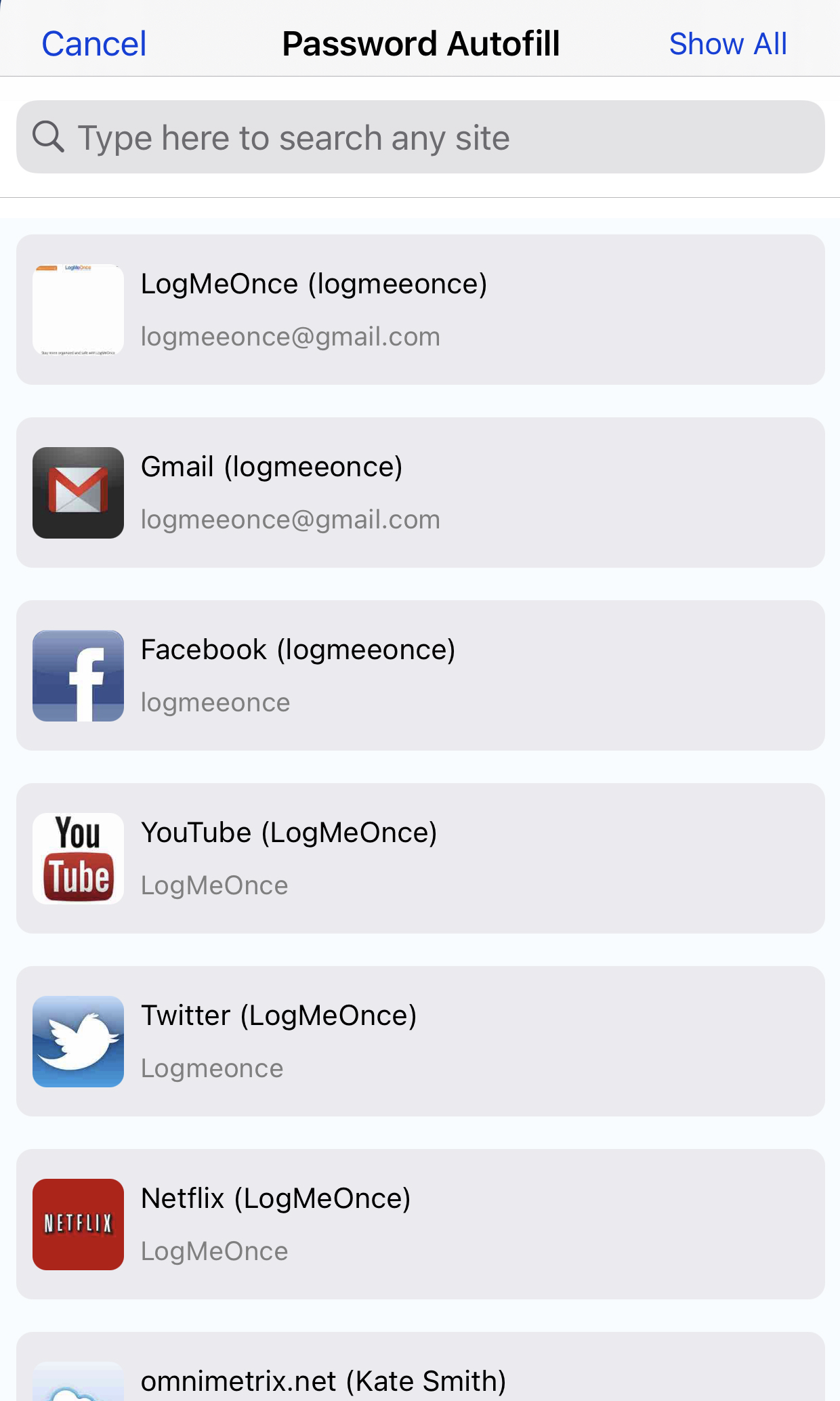The image displays an interface primarily divided into two sections. At the top, there is a light gray bar featuring two blue hyperlinks; "Cancel" on the left and "Show All" on the right. Centrally positioned within this gray bar is the label "Password Autofill" written in black text.

Beneath the gray bar is an interface with a white background, where a prominent light gray rectangular search box is located. This search box houses a magnifying glass icon on the left and contains the placeholder text "Type here to search any site."

Directly below the search box is a horizontal light gray line spanning the width of the interface. Under this line, there is a rectangular selection labeled "LogMeOnce," with the text "LogMeOnce" also appearing in parentheses. Below this, the email "logmeonce@gmail.com" is indicated.

Further down, another gray box appears, featuring a red and white envelope icon next to the text "Gmail: logmeonce@gmail.com." Below this, there is a blue Facebook icon followed by the text "Facebook (LogMeOnce)" and again "LogMeOnce." Lastly, a gray box at the bottom features a YouTube icon next to the text "YouTube: LogMeOnce."

This detailed caption thoroughly describes the elements and layout of the password autofill interface presented in the image.